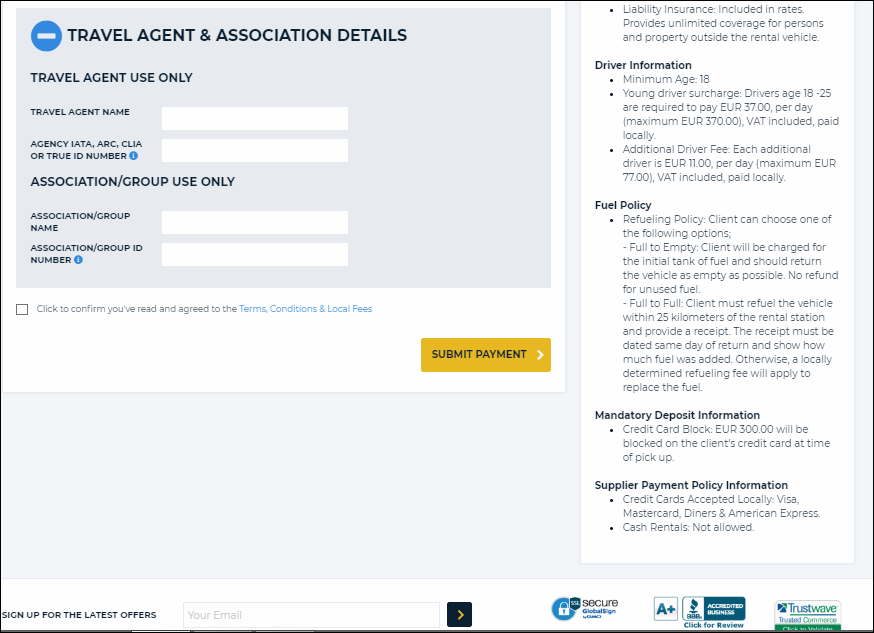The image showcases a detailed section of a car rental website's insurance and payment agreement page. In the upper-left corner, there is a gray box featuring a small circle with a minus sign. Below this, the page is divided into sections:

1. **Travel Agent and Associations Details**:
   - A heading for "Travel Agent Use Only" followed by fields for “Travel Agent Name,” “Agency ID,” “ARC, CLA, or True ID Number.” There is also a small blue information button next to these fields.
   - A separate section labeled “Association Group Use Only” containing fields for “Association Group Name” and “Association Group ID Number.”

2. **Terms and Conditions**:
   - A checkbox labeled "Click to confirm you've read and agree to terms and conditions and local fees," with the text "terms and conditions and local fees" highlighted in blue.
   - A yellow button with black text that reads "Submit Payment," accompanied by a forward arrow, positioned in the bottom right corner of this box.

3. **Insurance Agreement**:
   - The upper right section appears to cover the insurance agreement.
   - **Liability Insurance**: Includes limited coverage for a person’s property outside the rental vehicle.
   - **Driver Information**: 
     - Minimum age: 18.
     - A surcharge of EUR 37 per day (maximum EUR 370) for drivers aged 18 to 25, payable locally.
     - Additional driver fee: EUR 11 per day (maximum EUR 77), also to be paid locally.
   - **Fuel Policy**: 
     - Two options: full-to-empty and full-to-full.
     - Full-to-empty: The client pays for the initial tank, returning the vehicle as empty as possible, with no refund for unused fuel.
     - Full-to-full: Requires the client to refuel within 25 kilometers of the station, providing a dated receipt showing the added amount on the return date. A locally determined refueling fee applies if not adhered to.
   - **Mandatory Deposit**: 
     - A credit card deposit of $3,100 will be blocked at pickup. Accepted cards: Visa, MasterCard, Diners, and American Express. Cash rentals are not permitted, as this is likely illegal.
 
At the bottom of the image, a series of security badges, including an A+ rating and Trustwave Secure, certify the website’s safety.

Overall, this image describes a car rental website’s insurance page, with detailed terms and conditions regarding insurance, driver fees, fuel policy, and mandatory deposit requirements.